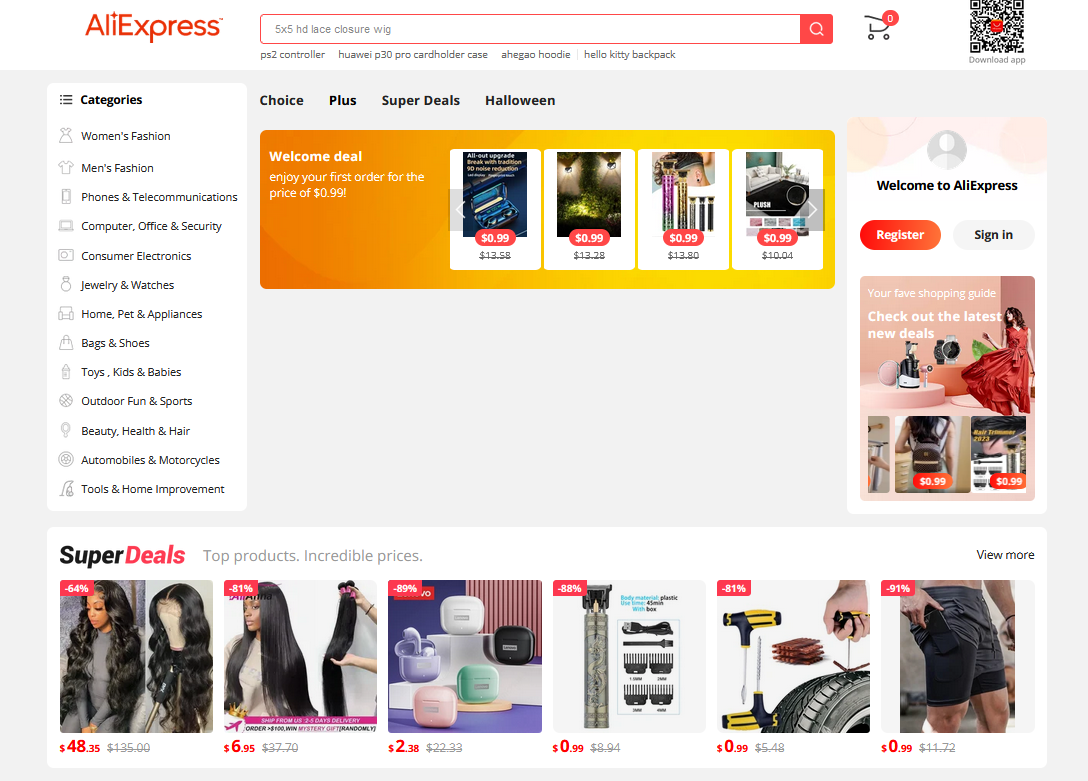This screenshot captures a vibrant and structured layout of the AliExpress homepage. Dominated by a bold, almost red-orange header, the page is organized into various sections. On the left-hand side, there is a 'Categories' menu icon depicted by three horizontal bars, listing a broad range of product categories: Women's Fashion, Men's Fashion, Phones & Telecommunications, Computer, Office & Security, Consumer Electronics, Jewelry & Watches, Home, Pet & Appliances, Bags & Shoes, Toys, Kids & Babies, Outdoor Fun & Sports, Beauty, Health & Hair, Automobiles & Motorcycles, and Tools & Home Improvement.

The right-hand side features an ad promoting a shopping guide with the message "Your Fave Shopping Guide, Check Out the Latest New Deals," highlighting deals for as low as 99 cents. Prominently visible is a QR code adorned with a red logo at the center, presumably for easy access via mobile devices. A search bar is situated at the top, pre-filled with the text "5x5 HD lace closure wig" in grey, exemplifying the type of product searches users can perform.

Further down, a welcome deal is advertised, offering users the opportunity to enjoy their first order for just 99 cents, along with various crossed-off items suggesting discounts. In another prominent section labeled 'Super Deals', six top products offering incredible prices are showcased, including a drill, men's shorts, and off-brand AirPods, reflecting the diverse range of affordable items available on the platform.